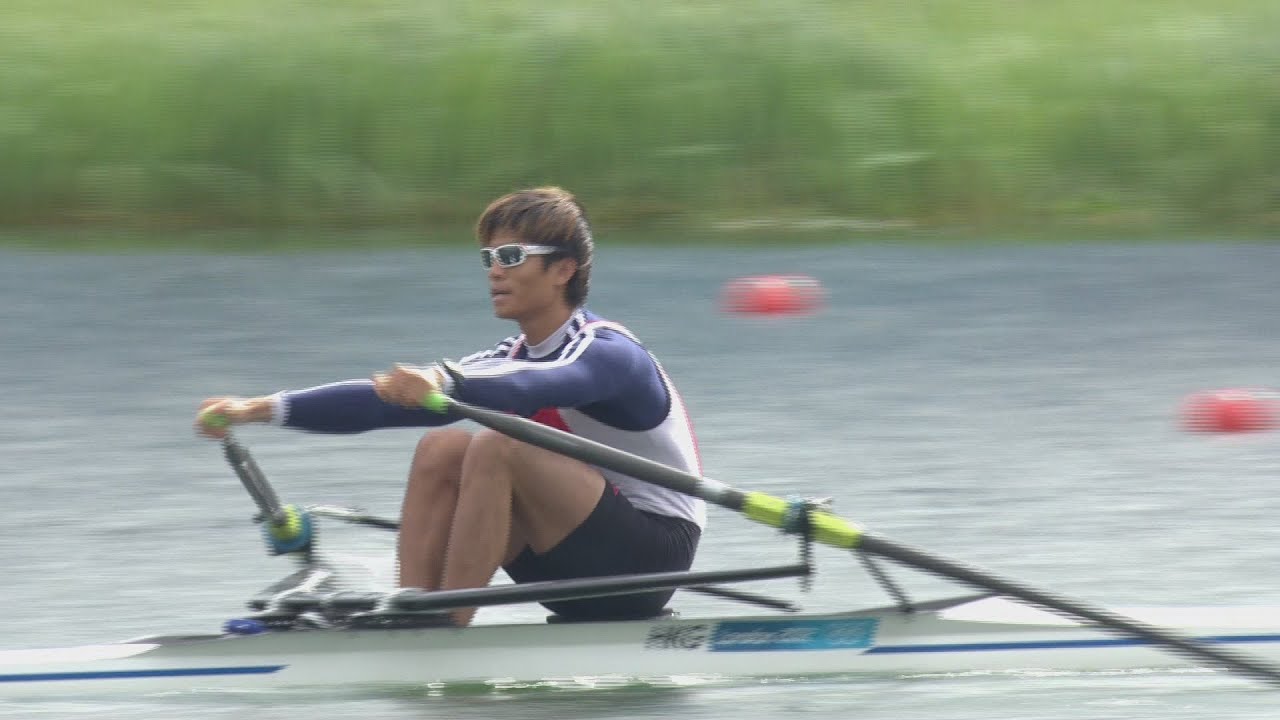In this dynamic photo, a singular rower is captured in mid-stroke, rowing at speed on a calm lake. The athlete, who appears to be of Southeast Asian or Indigenous descent, sports short, thick dark hair with possible brown highlights. He is dressed in a professional long-sleeved rowing uniform, featuring a blue and white top with black Lycra shorts. Silver sunglasses shield his eyes as he faces to the left, looking back towards where he has come from. His hands grip the oars that extend from a white rowing mechanism with blue stripes and unreadable lettering or numbers inscribed on its side. In the background, vibrant greenery and two red or orange buoys are blurred, emphasizing the rower's swift movement. The photograph is brightly lit, suggesting it was taken during the day. Yellow-wrapped sections are visible on the grey metal poles of his rowing setup. The athlete appears deeply focused, ready to execute a powerful stroke and propel himself forward.